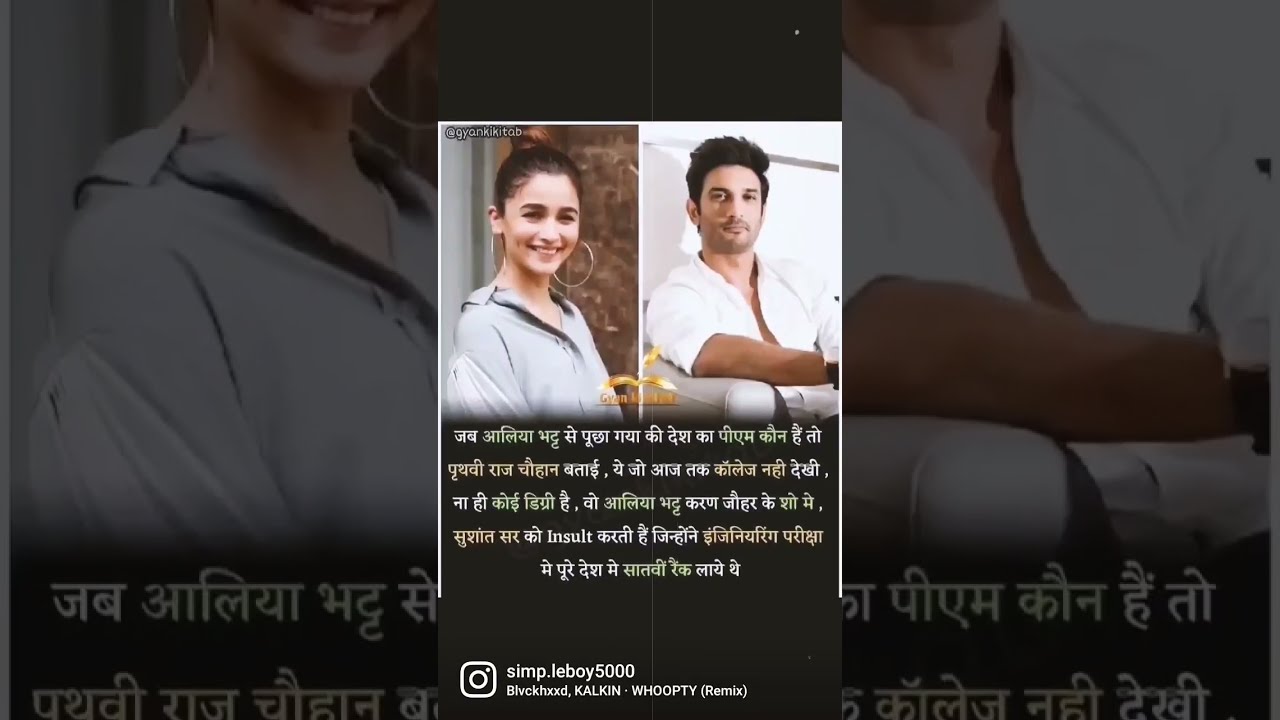In the center of the image, there are two people side by side—each prominently featured against distinct backgrounds. The woman, positioned slightly to the left of center, has her black hair pulled back into a bun. She wears an oversized, loosely-fitted blue collared shirt with the collar resting on her shoulders, and she's accessorized with giant gold hoop earrings, nearly the size of grapefruits. Behind her, through a window, one can discern some leaves, suggesting a natural setting. To her right and slightly off-center, the man sports thick, short black hair styled upward and a 5 o'clock shadow beard. He wears a white, short-sleeved collared shirt that is unbuttoned down the middle, revealing part of his chest. He rests his arm on what appears to be a white chair. Both individuals are set against different backgrounds: the woman against a leafy, light-colored backdrop and the man against a contrasting darker one. Below their images, which are side by side, there is a gray strip filled with unreadable text in a foreign language. Beneath this text, a Pinterest logo with the handle "simp.lboy5000" can be seen, followed by another unreadable text line with what looks like "blvckhxxd, calconwhooptyremix." Flanking this central image, the same photo of the man and woman repeats, much larger and cropped. On the right, the man’s face is cut off, only his neck and arm visible, and on the left, the woman's face is cut off, showing just the lower part of her face and her ear. This larger, repeated image extends into the background, taking up the outer thirds of the overall image.